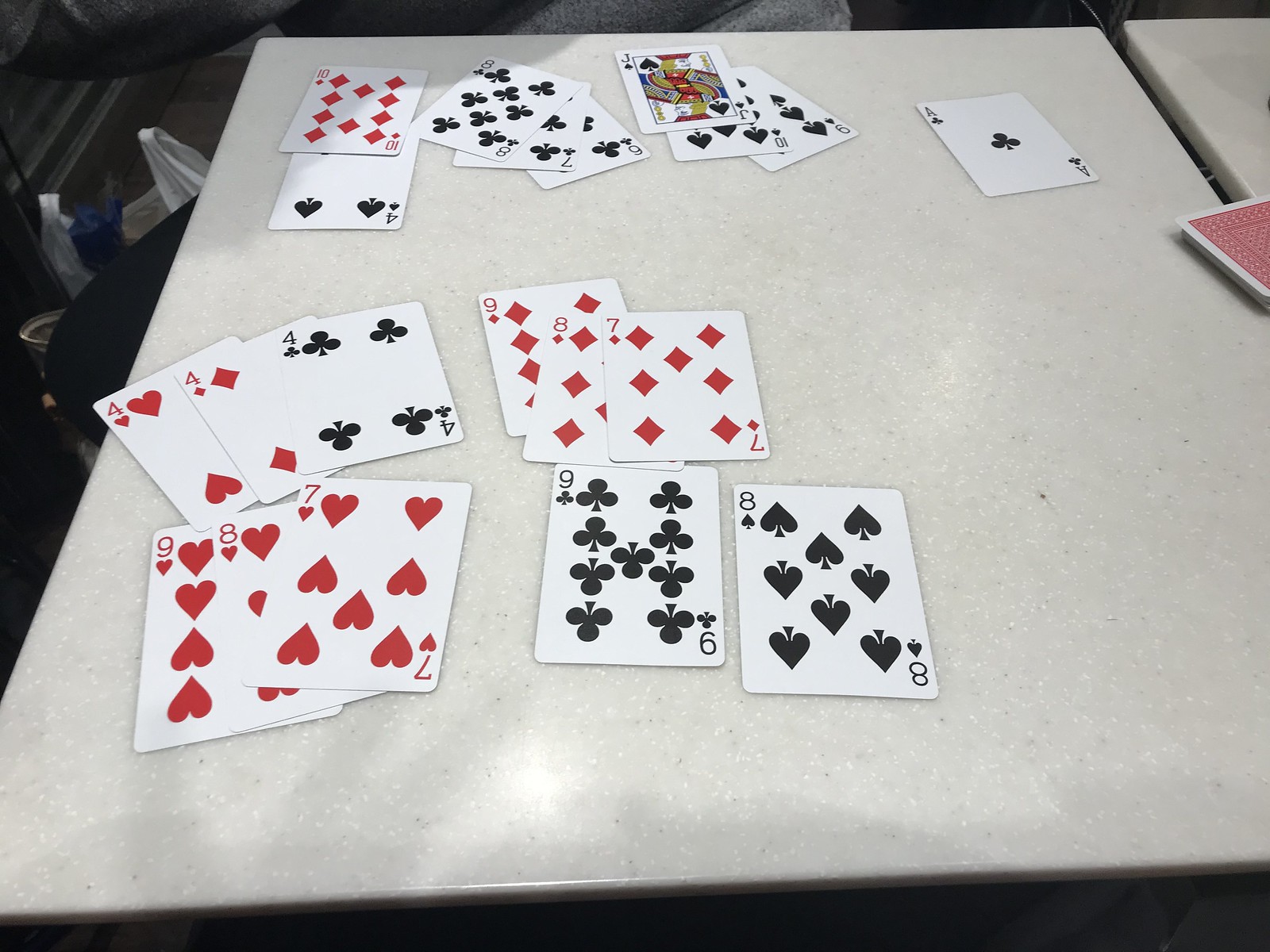In this detailed photograph, a card game is in progress on a large fold-out table. The table, which features a white top and black fold-down legs, is split down the center by a noticeable partition, though only the left-hand side is clearly visible in the image. The table surface is populated with 20 face-up playing cards, meticulously arranged in several rows, while the remaining cards are stacked face-down on the central partition.

In the bottom-most row, from right to left, the cards displayed are: 8 of Spades, 9 of Clubs, 7 of Hearts, 8 of Hearts, and 9 of Hearts. Moving upwards to the middle row, the cards, arranged from left to right, are: 7, 8, and 9 of Diamonds, followed by 4 of Clubs, 4 of Diamonds, and 4 of Hearts. The top row, from right to left, starts with a solitary 8 of Clubs, followed by the 9, 10, and Jack of Spades. To the left of these are the 6, 7, and 8 of Clubs, and then a 4 of Clubs with a 10 of Diamonds placed on top of it.

The setting of the photograph emphasizes the organized yet dynamic nature of the card game, with an interesting mix of suits and numbers showcased prominently on the table.